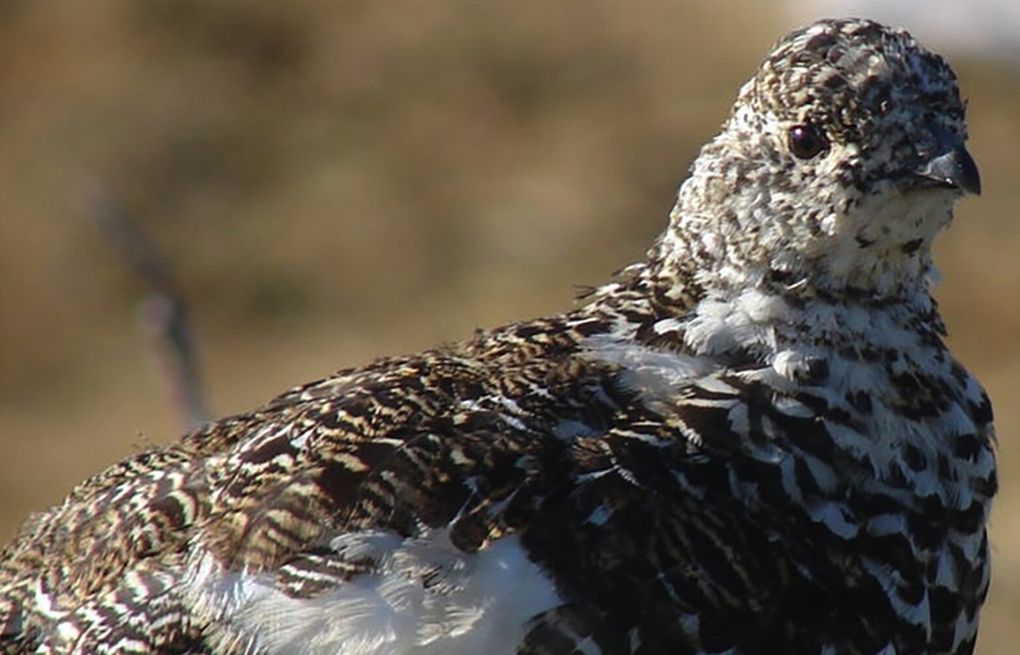This is a close-up color photograph of a bird, likely a grouse or a similar wild game bird, perched outdoors against a blurred brown background. The bird's head is on the right side of the image, revealing its tiny, pointy gray or black beak and beady black eyes. The bird's feathers are an intricate mix of white, brown, and dark brown, creating a fluffy appearance. Its head feathers predominantly display white with some interspersed darker hues. The chest area showcases a combination of white and brown stripy feathers, leading to a mostly brown body with lighter brown elements. Further down, a significant section of the bird's wings appears mostly white, indicating the wingtips. In the blurred background, indistinct gray, light brown, and green shrubs can be discerned, with a brown stick noticeable on the left-hand side.